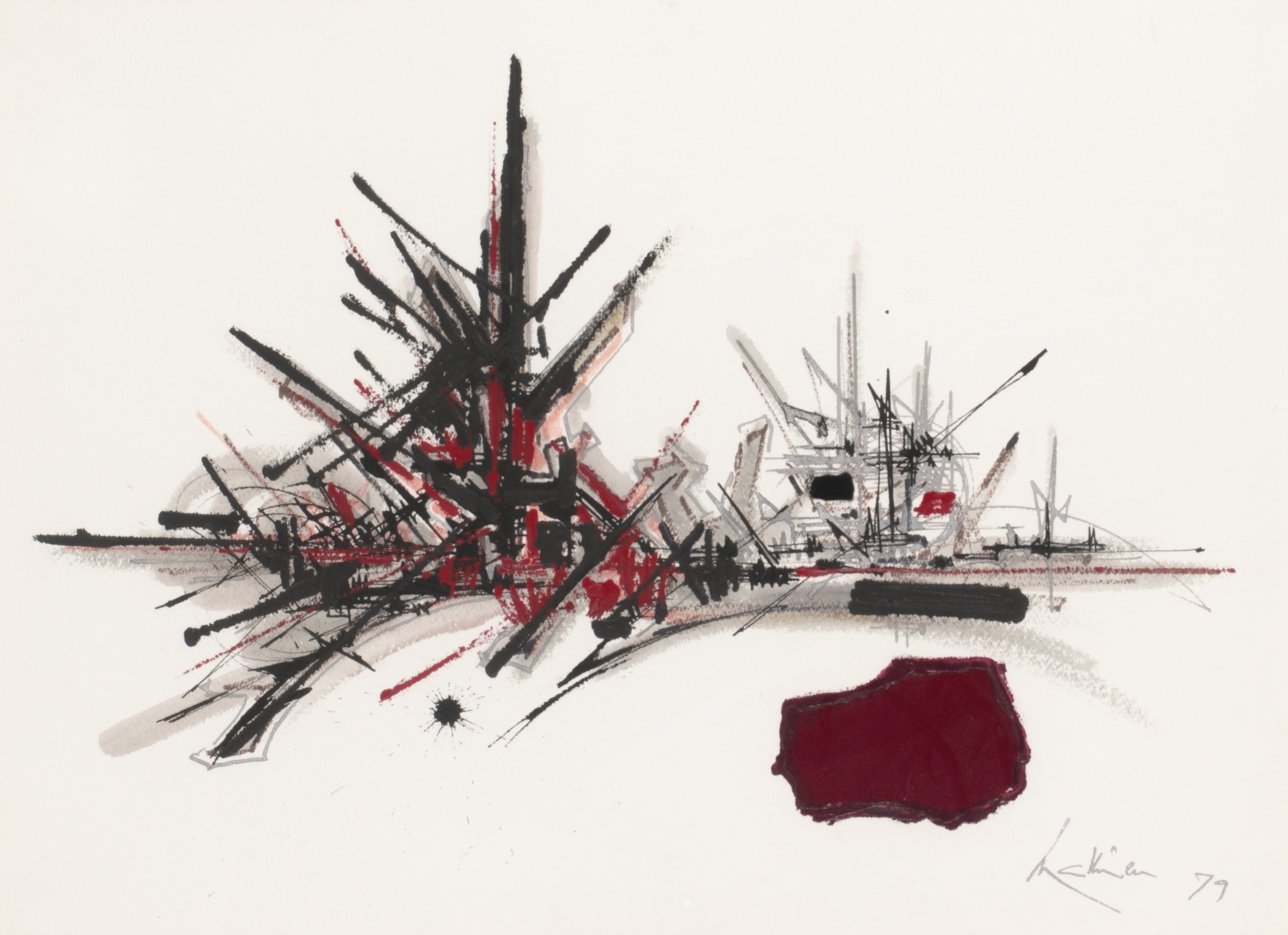The image is a wide rectangular painting with an off-white background, featuring a gray signature in the bottom right corner, dated either '71 or '79. Prominently in the foreground, a thin red line stretches horizontally across the center. Towards the left, several very thick black lines intersect in various directions, creating a pattern that's interspersed with black, red, gray, and light brown colors. These lines somewhat resemble abstract towers or structures. The background features faint, thicker gray lines and some light orange ones, adding depth. On the right side, there are fewer red elements but more thin gray lines accompanied by even thinner black lines. In the lower left corner, near the signature, there's a deep red splotch. The overall composition evokes a sense of organized chaos with a mixture of horizontal, vertical, and diagonal lines.